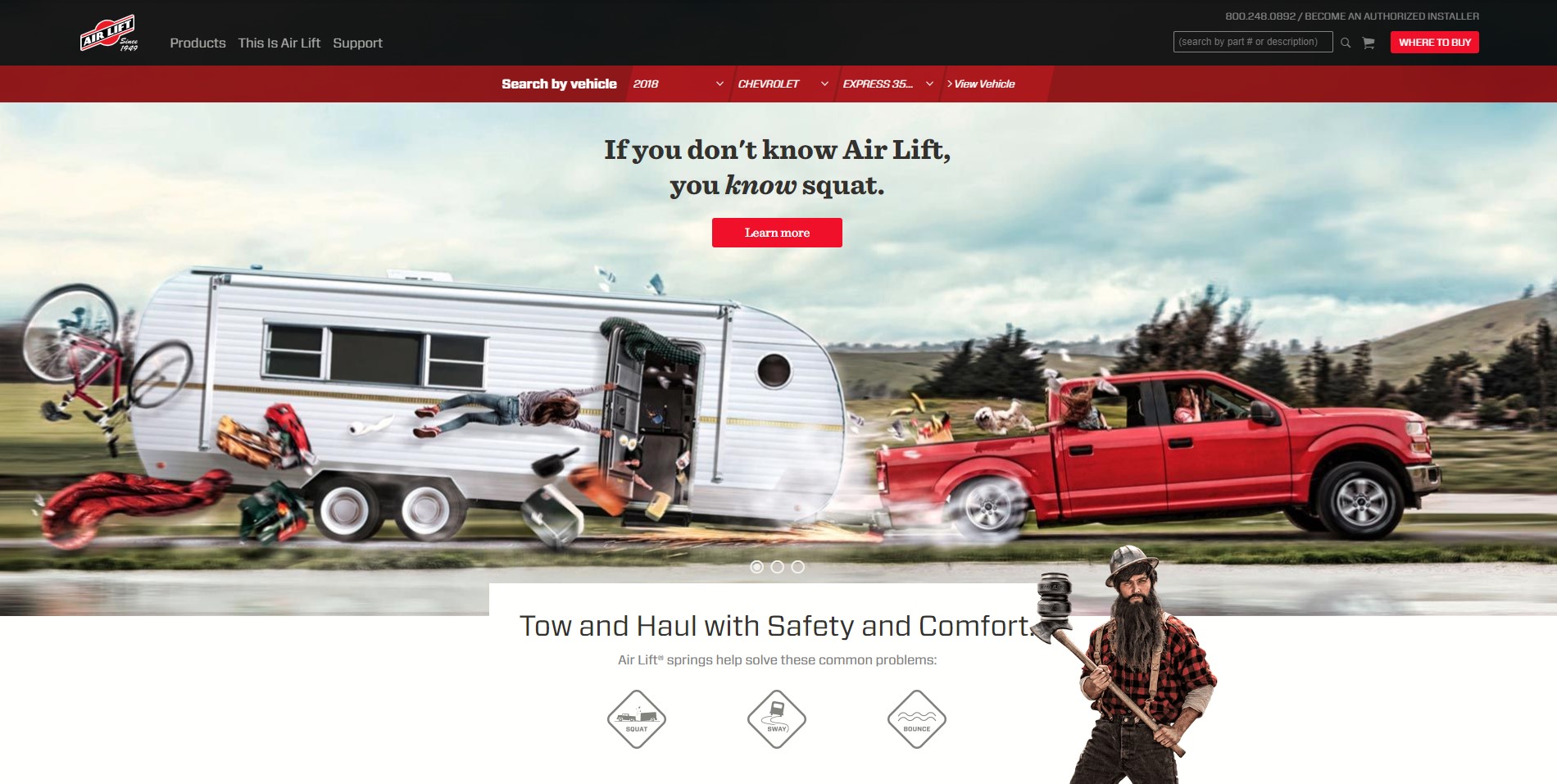The image is an advertisement for Airlift featuring a dramatic and chaotic scene. At the forefront, there is a prominently displayed tagline: "If you don't know Airlift, you know squat." The background showcases a heavily burdened four-door red truck towing an overloaded camper. The front end of the truck is scraping the ground under the excessive weight, highlighting the strain of the journey. Amid the commotion, a woman or child is seen clinging to an open camper door, flung outward and nearly horizontal due to the imbalance. Various items, including a bicycle, are depicted flying out of the camper, adding to the sense of disarray.

The bottom section of the advertisement reassuringly states, "Tow and haul with safety and comfort," suggesting that Airlift springs can mitigate such issues. It lists common problems solved by Airlift in a diamond-shaped area: "Squat, Sway, and Bounce." To reinforce the message, a rugged lumberjack figure holding an axe is featured, accompanied by a set of black Airlift springs, symbolizing strength and reliability.